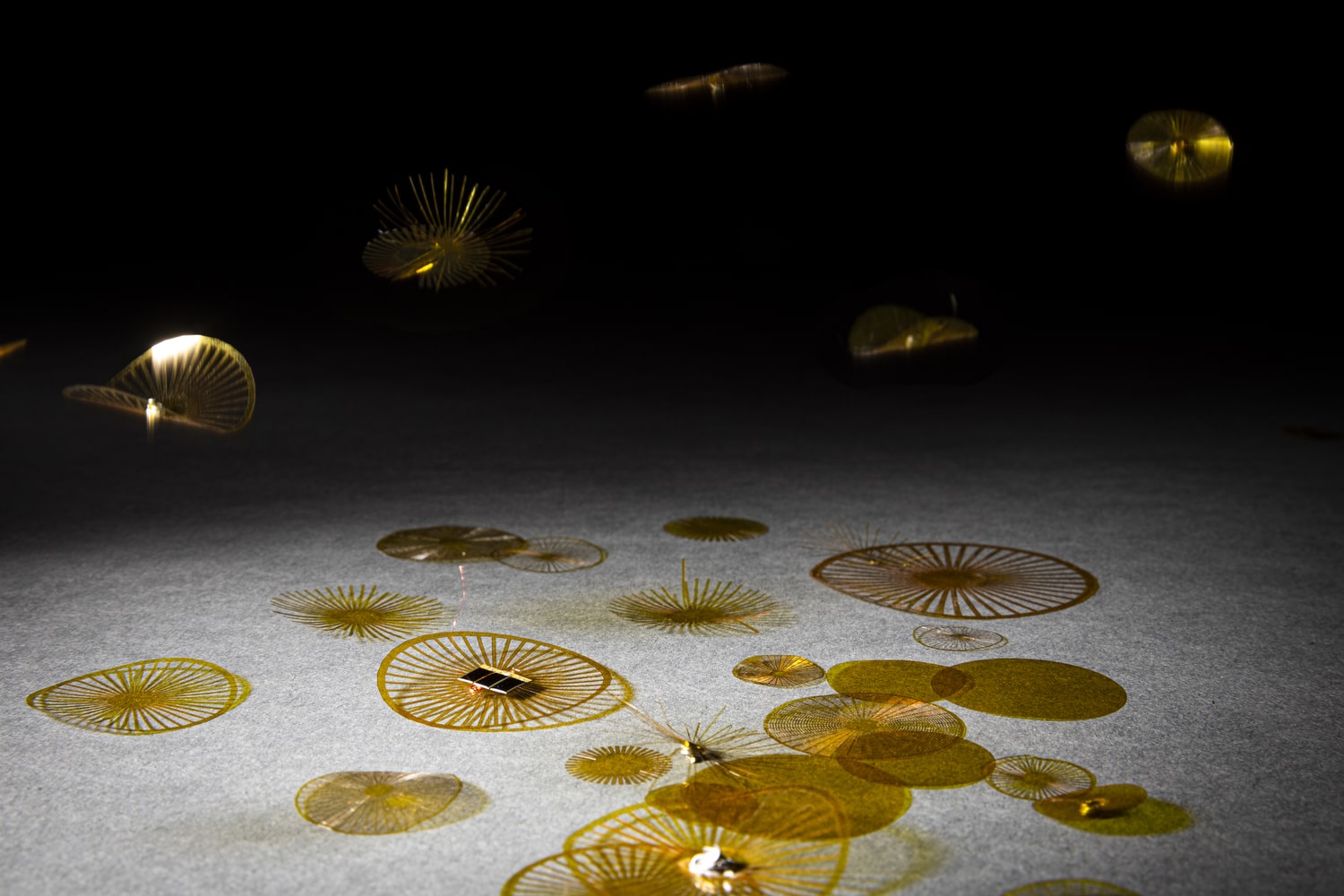The image showcases an indoor scene with multiple gold disks of varying sizes, some lying on a blue carpet and others floating in the air above. These disks, characterized by a radial pattern resembling the spokes of a wheel, exhibit a shiny golden-yellow color. The background towards the upper part of the scene is dark, while a light shines on the carpet at the front. Amongst the disks, there is a small, round object with long, thin, spider-leg-like filaments protruding from it. Some disks appear solid, while others have a see-through design. There's an impression that certain elements might be electronic, with insect-like objects perched on a few of the disks. The overall ambiance of the scene combines elements of ground and air, creating a surreal and mesmerising display of gold shapes against a contrasting backdrop.